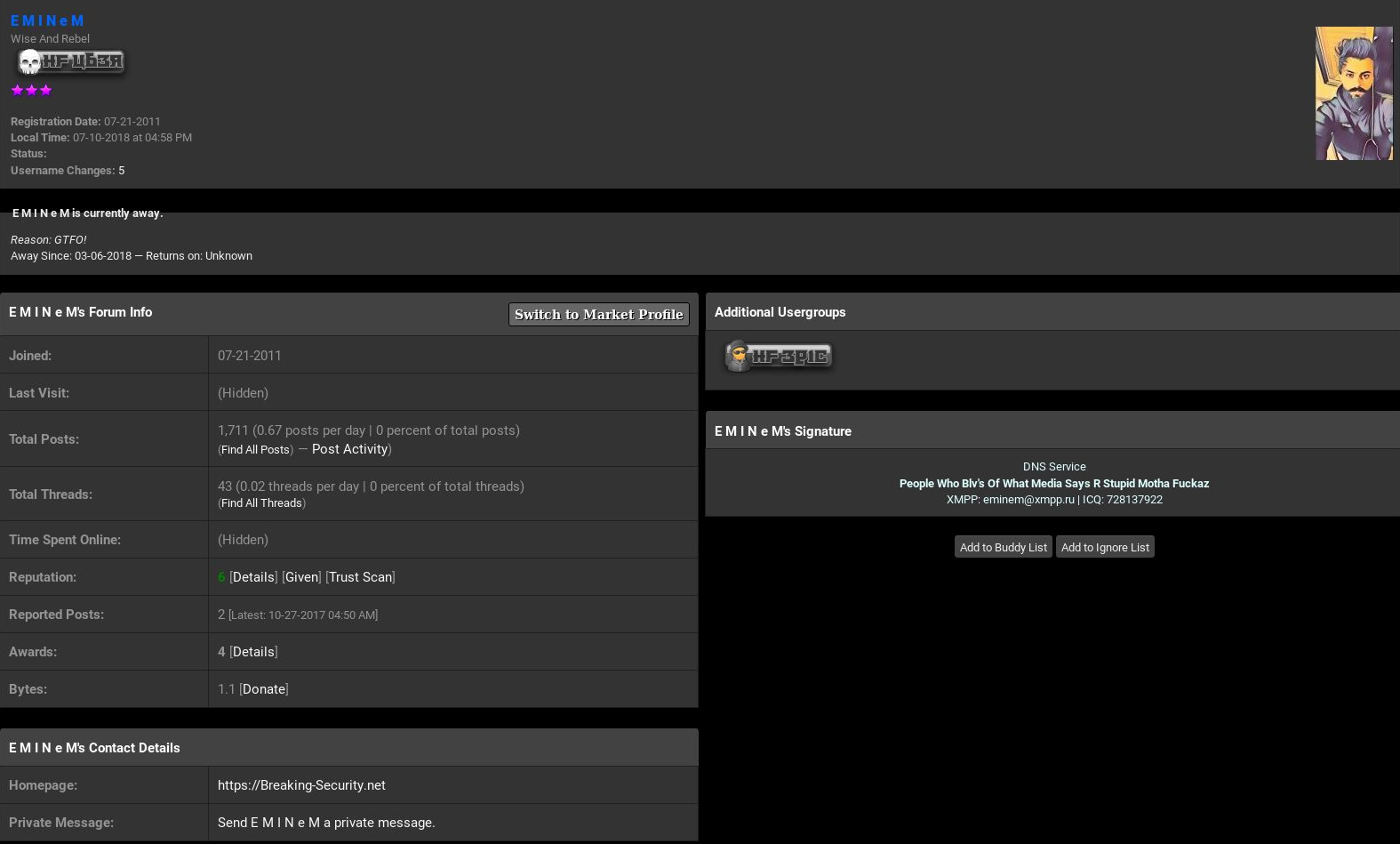**Caption:**

This is a screenshot of an admin panel from an online forum, possibly dedicated to or involving the handle "EM!NEM" (with the final "E" in lowercase). At the top, the name "EM!NEM" is prominently displayed next to a graphic consisting of a skull adorned with unusual characters and three pink stars below it. The panel indicates the user "EM!NEM" registered on July 21, 2011. 

Despite the blurriness of the image, certain statistics are visible: the user has made 1,711 total posts, participated in 43 threads, and has other metrics such as reputation, time spent online, reported posts, awards, and bytes listed. To the right of the panel is an illustrated image of a man wearing what appears to be armor and a beard, likely serving as the user's avatar.

Additional elements include some DNS service information, an area for adding a signature, and two unreadable buttons due to the low resolution of the screenshot. The background features a combination of light grey panels over a dark grey background, contributing to the overall aesthetic of the admin interface.